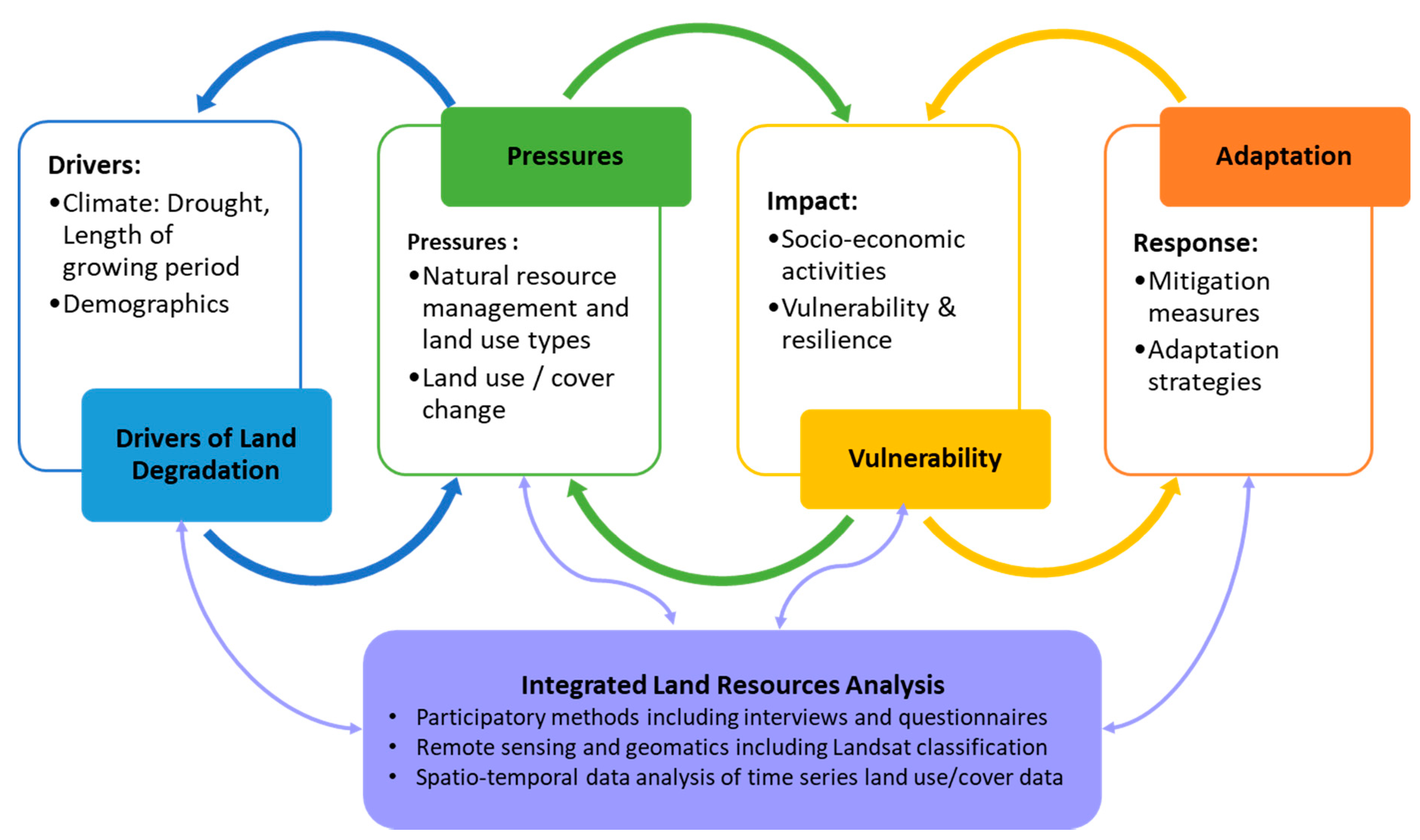The diagram, likely a part of a presentation or an academic report, provides a detailed analysis of integrated land resource analysis and its various components. It is color-coded and organized into four main sections represented by rectangles at the top: Drivers (blue), Pressures (green), Vulnerability (yellow), and Adaptation (orange). 

The Drivers section includes factors such as climate, drought, length of the growing period, and demographics. The Pressures section addresses aspects like natural resource management and land use types, as well as land use and cover changes. The Vulnerability section discusses socioeconomic activities, resilience, and the overall impacts. The Adaptation section focuses on mitigation measures and strategies for adaptation.

Beneath these four sections is a purple rectangle labeled "Integrated Land Resource Analysis," which includes participatory methods such as interviews and questionnaires, remote sensing and geomatics like Landsat classification, and spatio-temporal data analysis of time series land use/cover data. Color-coded arrows connect these sections, indicating the flow and relationship between Drivers, Pressures, Vulnerability, and Adaptation, with the integrated land resource analysis synthesizing these aspects. The diagram is vibrant and detailed, making complex interrelations clear and visually accessible.